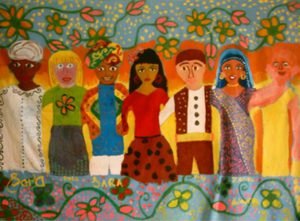The image is a horizontally aligned, rectangular painting depicting seven diverse figures assembled closely together. Each character exhibits distinct cultural attire and features. On the far left, a black man wears a white hat and a white gown, reminiscent of a dashiki or a Bombay-style suit. Next to him stands a blonde woman with a playful expression, dressed in a green top adorned with a flower and a gray skirt. Beside her, a dark-skinned individual with floral decorations on a colorful ornate hat sports a blue shirt with multicolored sleeves and white pants. The central figure is a Hispanic-looking woman with a serious expression, long black hair, and bangs; she is clad in a red top and a polka-dotted dress or skirt. To her right stands a man in a brown vest over a white shirt and brown pants, featuring a yellow belt and what might be a bandana or do-rag on his head. The next figure is a woman in Indian-style clothing, with darker skin, gold earrings, and a blue veil. Finally, the rightmost figure, another woman, has vibrant blue hair and a warm smile. The background of the painting features a greenish-gray hue, adorned with coral, yellow, and green flowers, and interwoven vines, providing a lush frame to the diverse assembly.